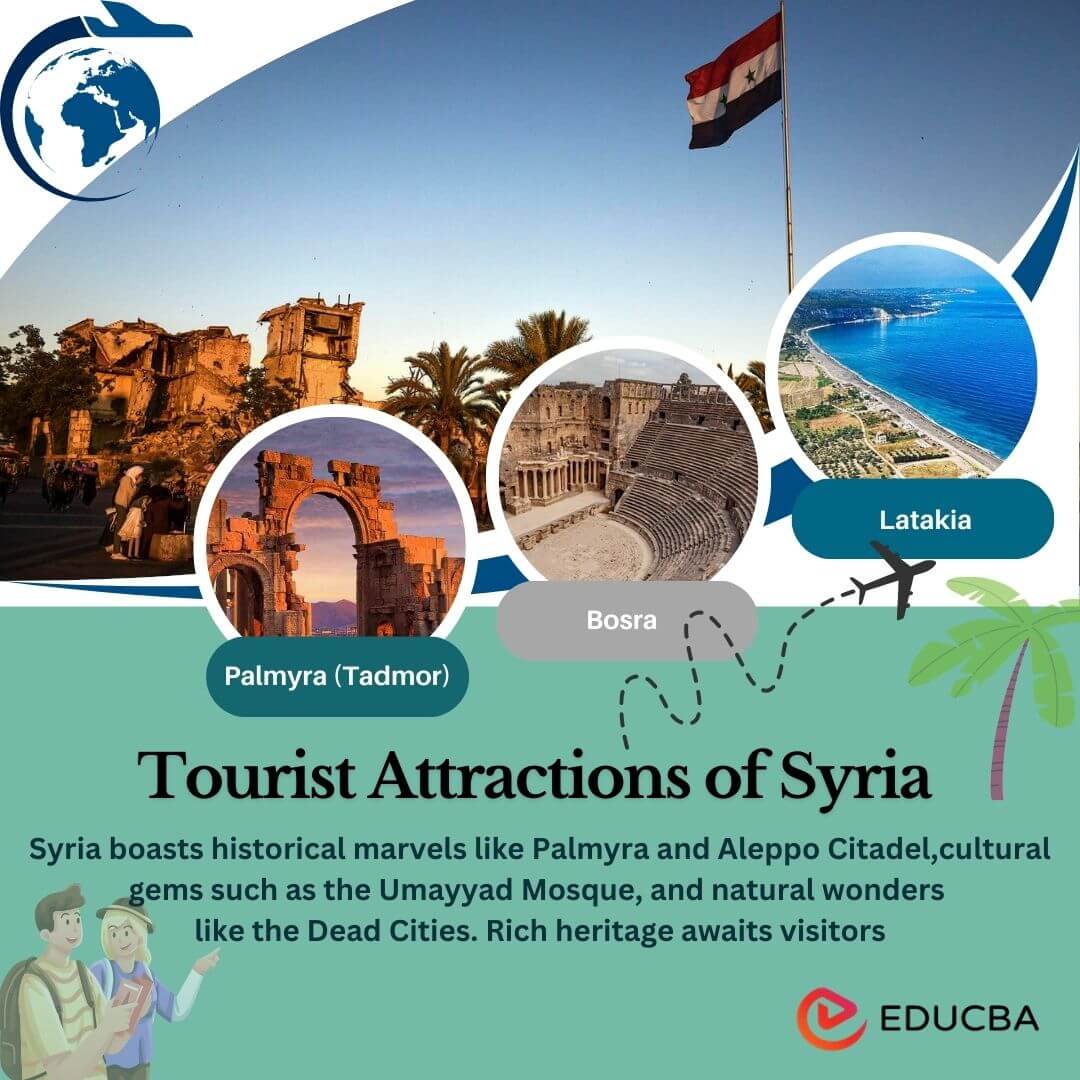This image is a detailed advertisement for the tourist attractions of Syria, potentially for a travel magazine or website. The top half features a colorful photograph of Syria’s landscape, showcasing beige stone buildings, palm trees, and a clear blue sky. A flag with red, white, and black stripes, and two green stars is visible on the right. In the center, three prominent circles highlight key tourist destinations: Palmyra (Tadmor), depicted with its famous stone archway; Bosra, showcasing an ancient stone stadium; and Latakia, illustrating its stunning seaside with vibrant blue waters.

The bottom half of the advertisement is a green text box with black ink that provides a detailed description: "Tourist attractions of Syria. Syria boasts historical marvels like Palmyra and Aleppo Citadel, cultural gems such as the Umayyad Mosque, and natural wonders like the Dead Cities. Rich heritage awaits visitors." Additionally, the bottom right corner features the name "EDUCBA," likely the proponent of this ad, while the bottom left corner showcases sketched figures of a man and woman along with a palm tree illustration. This intricate composition seamlessly blends Syria’s rich historical, cultural, and natural offerings, inviting travelers to explore the country's diverse heritage.